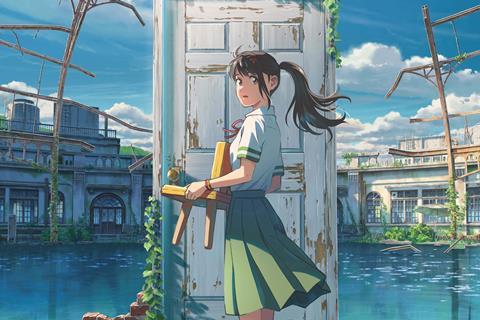In this detailed still from an anime-style show, a female character, likely a Japanese school girl, is centrally positioned in front of an aged, weathered exterior door adorned with a gold doorknob and shabby chic white chipped paint. Her black hair is styled in a ponytail with bangs and some loose strands hanging down in front of her ear. She makes eye contact with the viewer, her face turned three-quarters profile while her body remains in profile. She wears a traditional school uniform featuring a white collared short-sleeve shirt with two distinctive green stripes on each cuff, a red ribbon tied in a bow around her neck, and a green pleated skirt that reaches her knees. Additionally, she sports a brown watch on her left wrist.

In her hands, she carries a small yellow chair with short wooden legs. The backdrop reveals a dilapidated outdoor scene with a body of water directly behind her and an old door seemingly leading to nowhere. Surrounding the door are traditionally Japanese one-story buildings, some dilapidated electrical lines, and bits of ivy creeping up the left side and right corner of the door. The sky above is a vibrant blue with animated, cartoon-style clouds, creating a contrastingly serene atmosphere overshadowed by the evident partial destruction in the surroundings. Her expression appears worried, further evoking a sense of underlying tension and mystery in the scene.